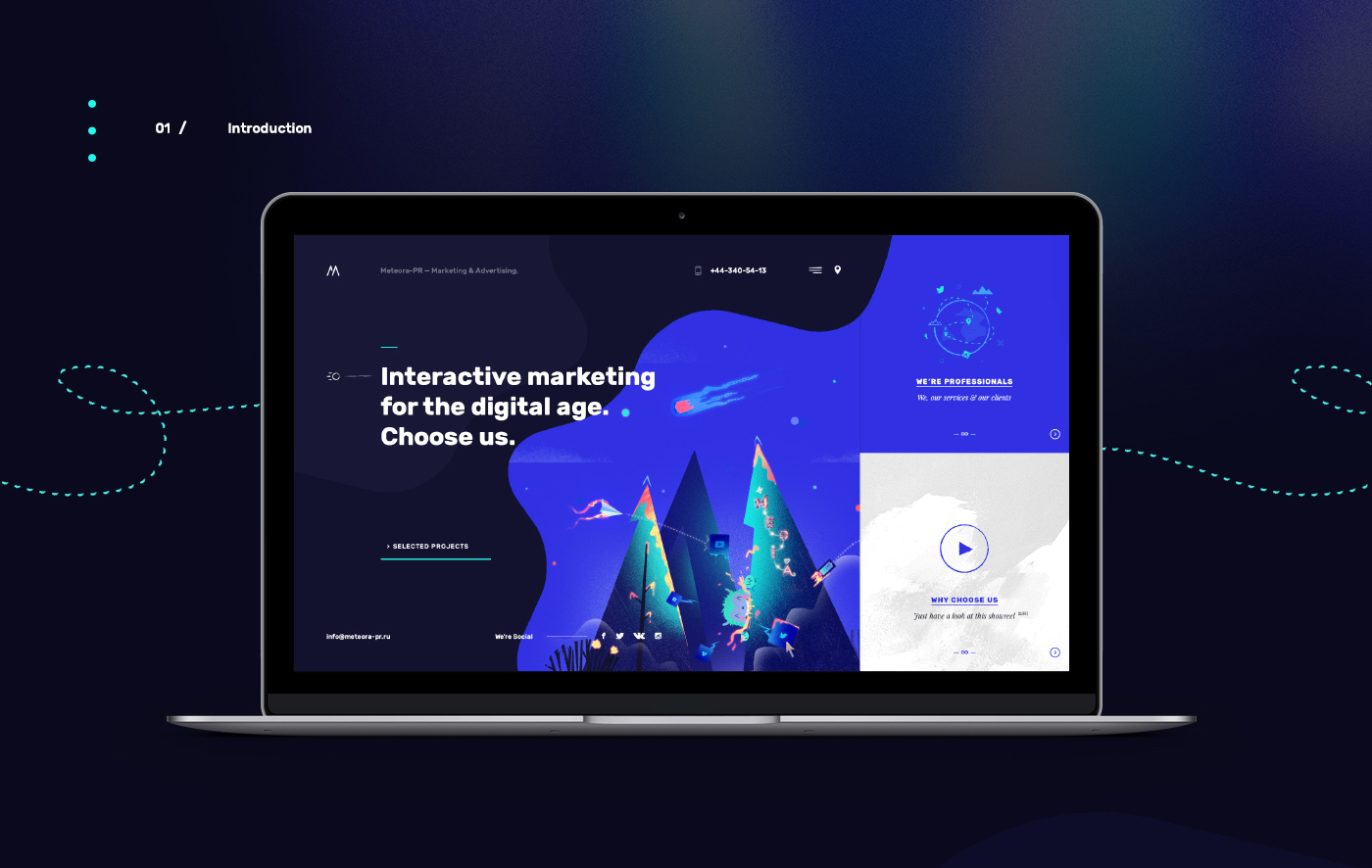The image features a black rectangular background. Within this black rectangle, there's a light blue-outlined smaller rectangle that also maintains the black background. Centered within this outlined rectangle is white text that reads, "Interactive Marketing for the Digital Age, Choose Us."

To the side of the text, there is a dark blue curvy outline of a small square. On a hill within the image, there are various colored trees, reminiscent of Google’s colors—red, yellow, green, and blue. Each tree contains tiny icons that are too small to discern clearly. Surrounding these trees are light blue squiggly shapes.

At the bottom right corner of the image, there is a white-outlined square play button within another light blue square. This play button is accompanied by some unreadable blue and black text due to its small size.

At the top of the black rectangle, there are three aqua green dots followed by the text "01/Introduction" in aqua. A dotted line in aqua starts at the left side of the image, then breaks upon reaching the central light blue rectangle, and resumes at the other end of this rectangle, continuing to the right edge of the black rectangle.